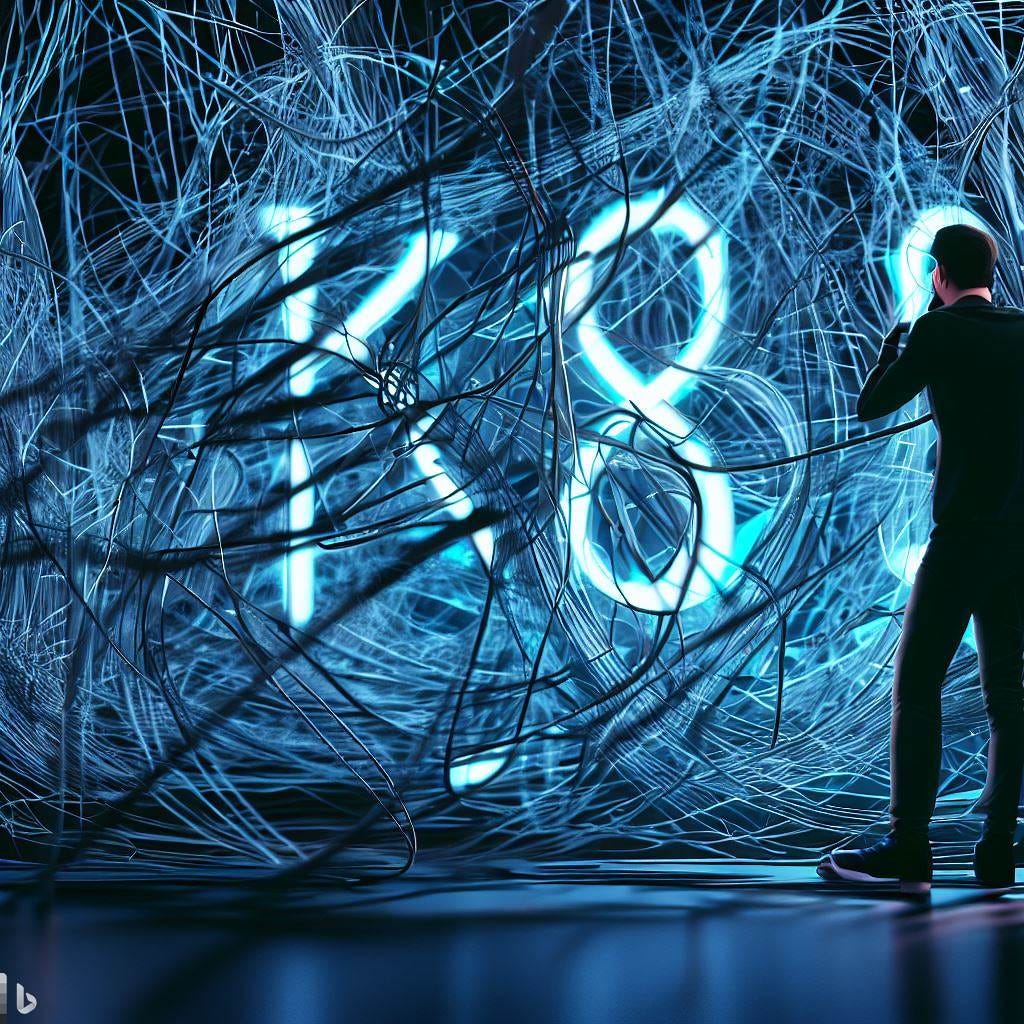The computer-generated image features a large, complex mass of hundreds of entangled, blue-lit wires dominating the scene. Situated in the midst of these wires are glowing, fluorescent white characters, "K8", which illuminate their surroundings with a neon-like glow. On the bottom left corner of the image, there's a small watermark resembling the Bing logo. To the right-hand side, a man dressed entirely in black, including black sneakers with a distinct white stripe underneath, stands observing the luminous characters through what looks like a porthole, indicating a museum or gallery setting. The image has an overall blue hue, with the ground covered in a dark laminate floor that reflects the light from the glowing characters, enhancing the surreal, abstract quality of the artwork.